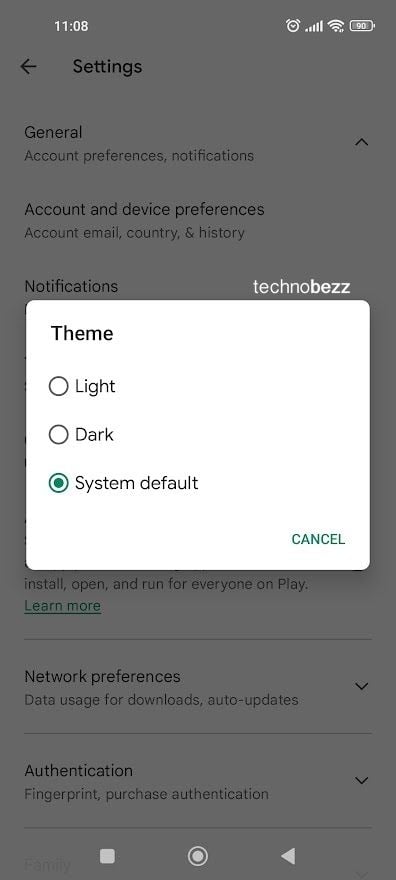Screenshot of a smartphone displaying a settings interface with a pop-up menu.

At the top of the screen, standard phone icons are visible. On the top right corner, a battery icon shows 90% charge, while icons for WiFi, cellular data connection, and an alarm clock are also present. On the top left, the time reads 11:08 AM.

The main display shows a grayed-out settings page with various menu options partially obscured by a white pop-up rectangle. The background settings include categories such as General, Account Preferences, Notifications, Account and Device Preferences (with sub-options like Account Email, Country, and History), and Network Preferences (covering areas like Data Usage for Downloads, Auto-Updates, and Authentication with fingerprint and purchase authentication).

The pop-up rectangle, centered on the screen, presents a theme selection menu titled “TechnoBez” at the top right corner of the rectangle. This menu offers three theme options: Light, Dark, and System Default, with the "System Default" option selected, indicated by a green-filled circle.

At the bottom right of the pop-up menu, there's a "Cancel" button. This pop-up is positioned directly below the "Notifications" section, obscuring some of the background settings text.